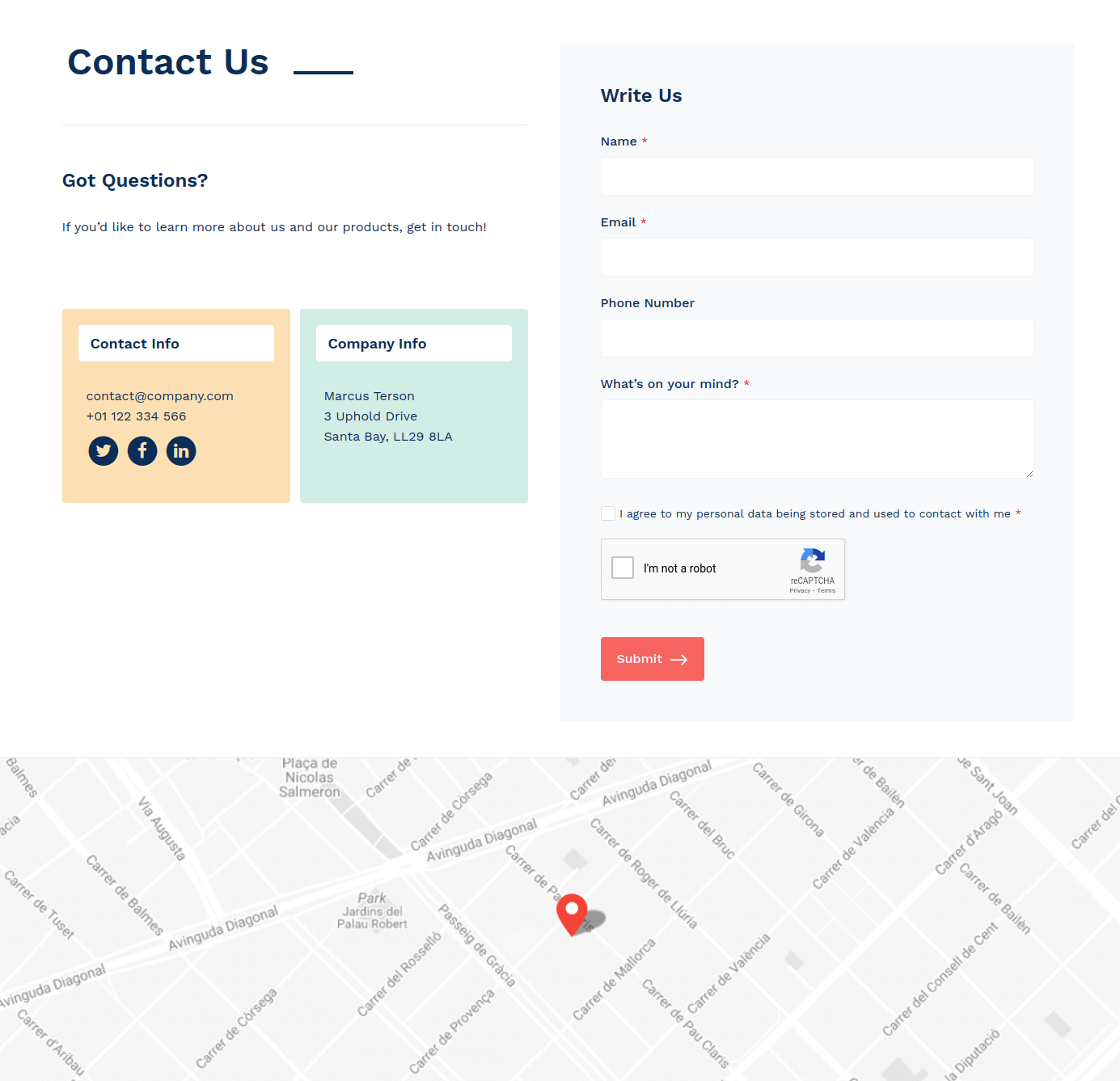The image depicts a "Contact Us" page on a website. The "Contact Us" heading is positioned in the upper left corner, highlighted in bold, black font, accompanied by a black underscore. Below this, a horizontal line divides the header from the subsequent content.

The first section poses the question, "Got questions?", followed by a line that reads, "If you'd like to learn more about us and our products, get in touch." Beneath this prompt are two prominent rectangular boxes. The left box, labeled "Contact Info" in bold text, is enclosed within a larger, approximately ten-shaded frame. Adjacent to it is another white rectangular box labeled "Company Info" against an aqua green background.

To the right, there's a faded gray box titled "Write Us," stretching across more than a quarter of the page's width. This section contains a field for "Name" marked with a star, indicating a required input, followed by a long white input box. Below it is another required field for "E-mail," also marked with a star, with an accompanying white input box. Additional fields include a "Phone Number" box and a "What's on Your Mind" text area, allowing users to detail their inquiries. 

At the bottom of the form, there is an “I’m not a robot” CAPTCHA verification, designed to prevent automated submissions. Below the form is an embedded map featuring a red location beacon in the center, indicating the company's address or point of contact.